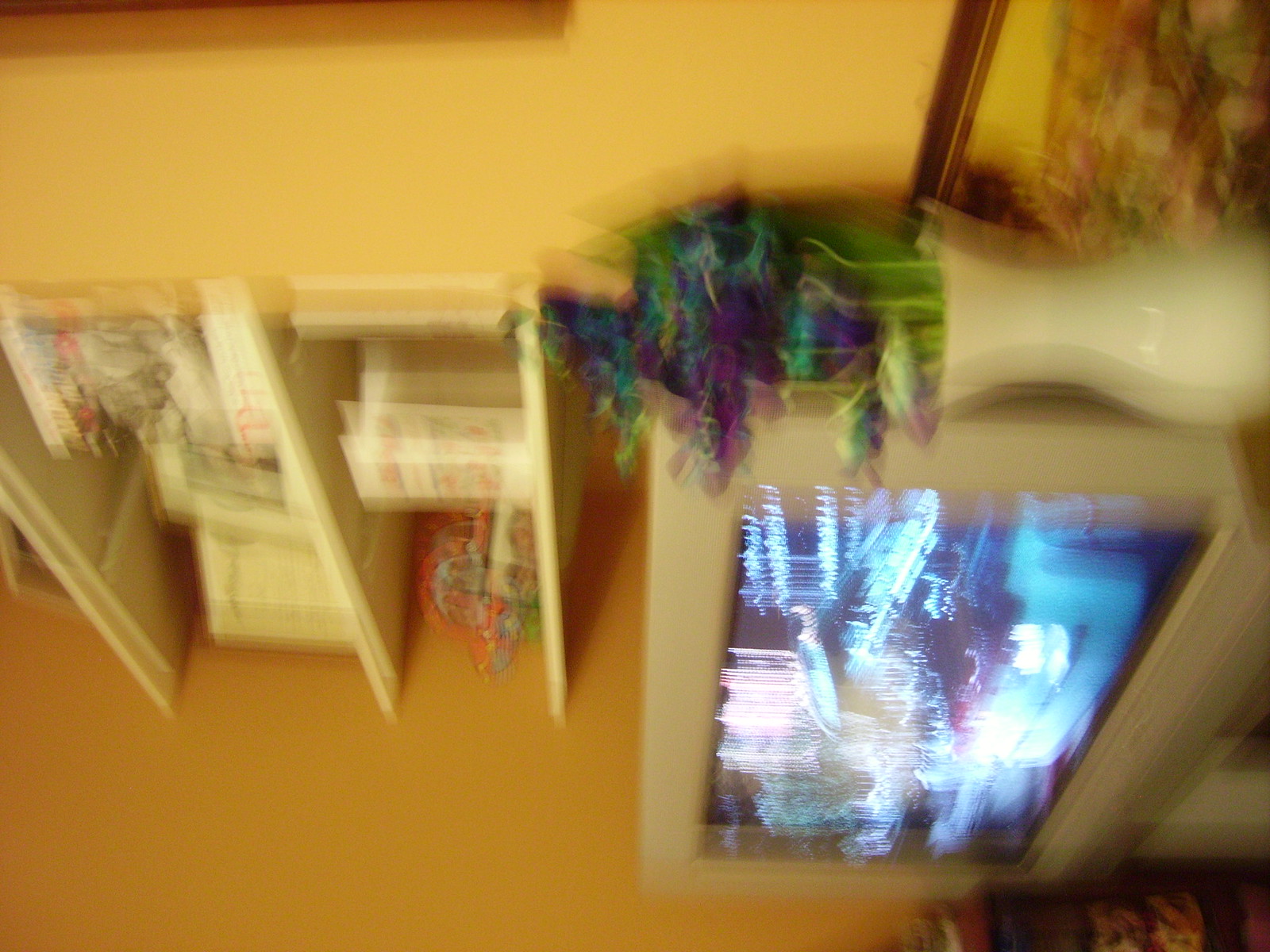This image depicts a disoriented and blurry photograph of a living area, taken in portrait but displayed landscape, making it difficult to discern details. The photo is rotated 90 degrees to the left, causing the left-hand side to appear closer to the ceiling and the right-hand side closer to the ground. Featured prominently is an old silver-framed CRT television displaying an indistinct image with streaks of white, black, green, orange, and blue. Beside the TV sits a distinctive white ceramic vase with a flared top, containing flowers that are purple, green, and blue, which might be artificial. The background showcases yellow walls, though the exact hue is indistinguishable due to the blur. Set into the wall are white shelves holding various décor items, including books, possible framed pictures, and what seems to be a child’s drawing of a car. The overall image is highly blurred and turned on its side, adding to the disorientation.